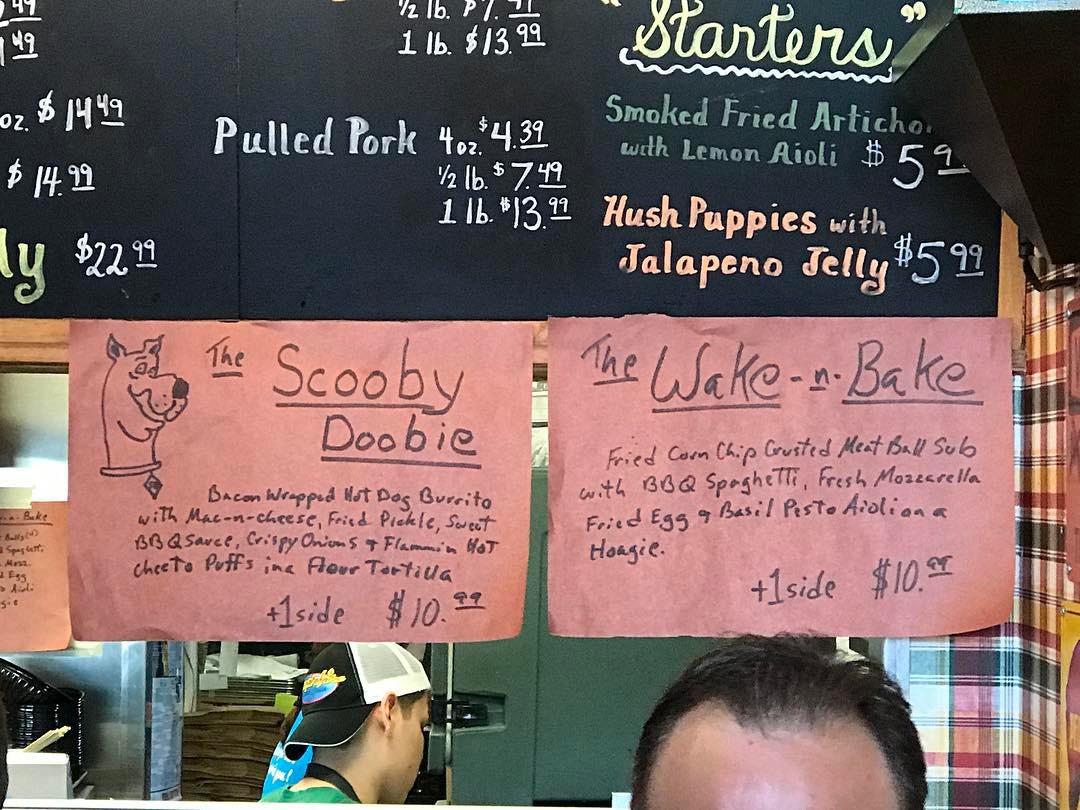This photograph captures a vibrant and bustling scene at a restaurant counter. The primary focus is a large blackboard menu hanging high above the ordering area, featuring an eclectic mix of handwritten items in chalk. The blackboard lists enticing options, including pulled pork available in portions of four ounces, half a pound, or one pound. The Starters section highlights smoked fried artichokes served with lemon aioli and hush puppies accompanied by jalapeño jelly.

Below the blackboard, two red pieces of paper with menu items handwritten in marker add a splash of color and informality to the display. One of these red papers showcases a playful drawing of a dog and features an item called the "Scooby Dooby," described as a bacon-wrapped hot dog burrito stuffed with mac and cheese, fried pickles, and other delicious toppings, priced at $10.99. Beside it, another item titled "Wake and Bake" is mentioned, hinting at another creative dish.

In the foreground, the top of a customer's head can be seen, as well as the back of an employee’s head, who is working diligently behind the counter in the kitchen area. This worker wears a green shirt and a hat turned backward, adding to the casual and comfortable atmosphere of the place. The backdrop reveals restaurant equipment like refrigerators and other kitchen essentials. On one side, red and green curtains frame a window, adding a cheerful and festive touch to the environment.